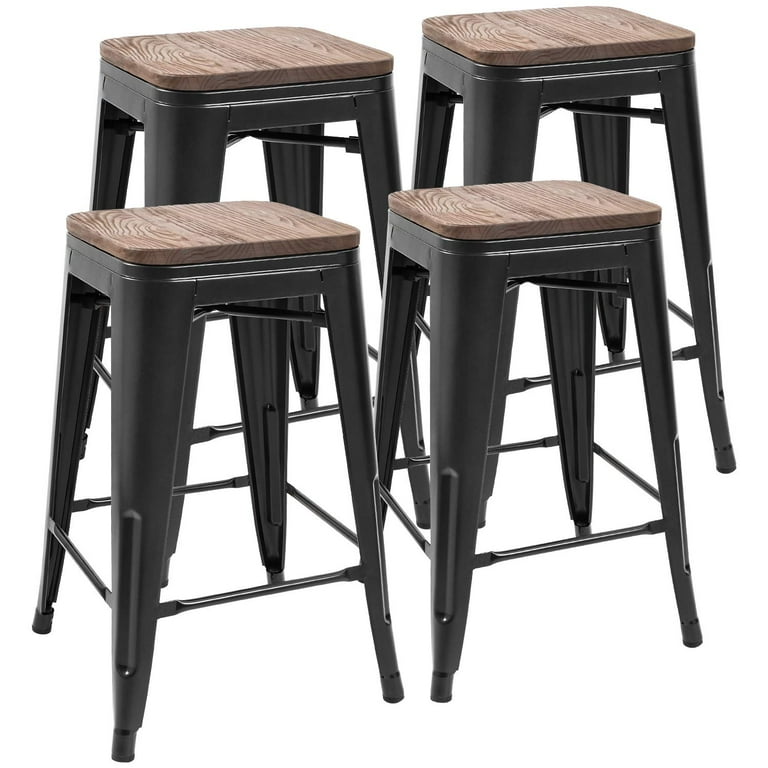In the image, there are four stackable stools arranged diagonally, from the lower left corner to the upper right. These stools feature a contemporary post-industrial modern design, ideal for a bar or kitchen setting. The tops are a matte, deep yet light brown wood with visible grain and knots, giving them an almost unfinished appearance. Each stool's edge is smoothly curved. The legs and supports are black metal, splaying outward until they touch the ground, forming an X-shaped reinforcement just beneath the seat. The metal legs are connected by rods welded into a square at the base, enhancing stability. The background is entirely white, with no shadows, giving the impression of a filtered image. The stools in the back row appear higher but are likely the same size as those in the front, suggesting different perspectives rather than actual size variation.